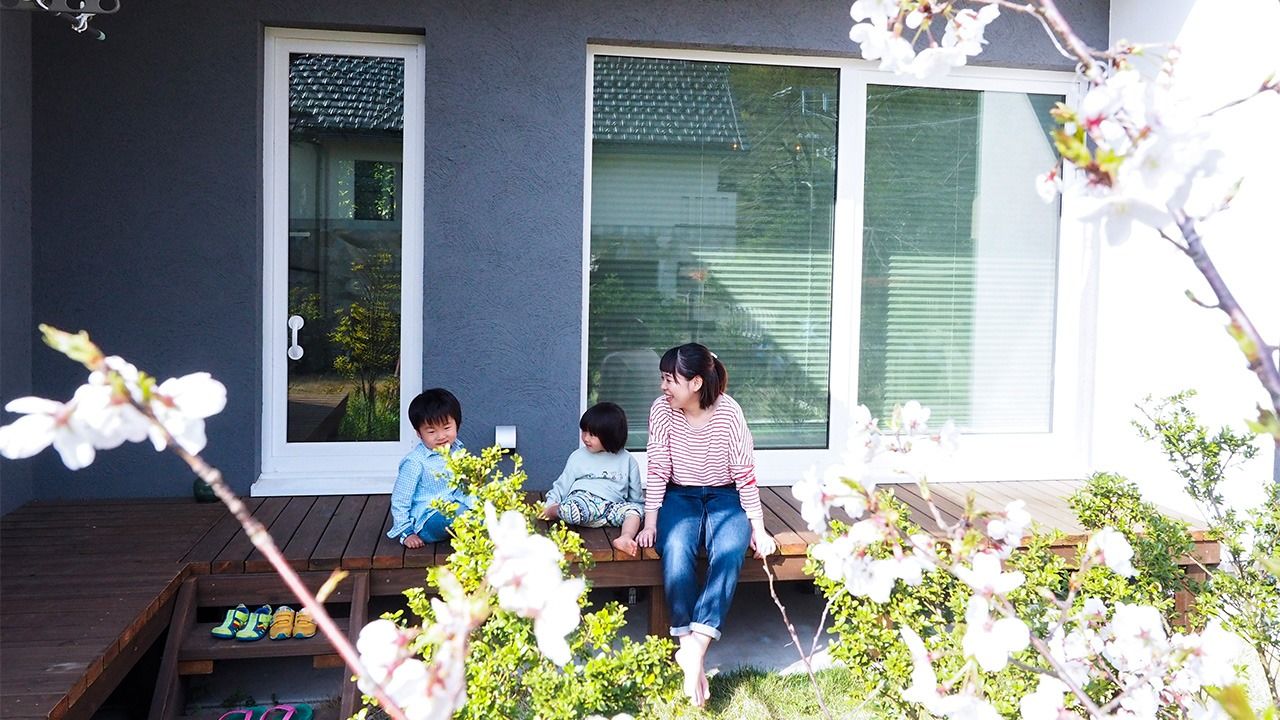A serene daytime photograph captures an Asian mother and her two small children seated on the wooden porch of their modern, blue stucco home with white trim. The mother, dressed in blue jeans and a red striped shirt, gazes lovingly at her young son to the left. The boy, with short brown hair, is clad in a long-sleeve blue shirt and blue jeans. Next to the son sits his sibling, and all three family members share dark hair and joyful expressions. The house features a white door with a glass body and two windows with blinds, adding to its simple yet contemporary charm. The L-shaped deck is connected to the ground by wooden steps, where two small pairs of children's shoes rest atop the step. The scene is framed by cherry blossom bushes and plants with delicate white flowers, enhancing the peaceful family moment amidst nature's beauty.